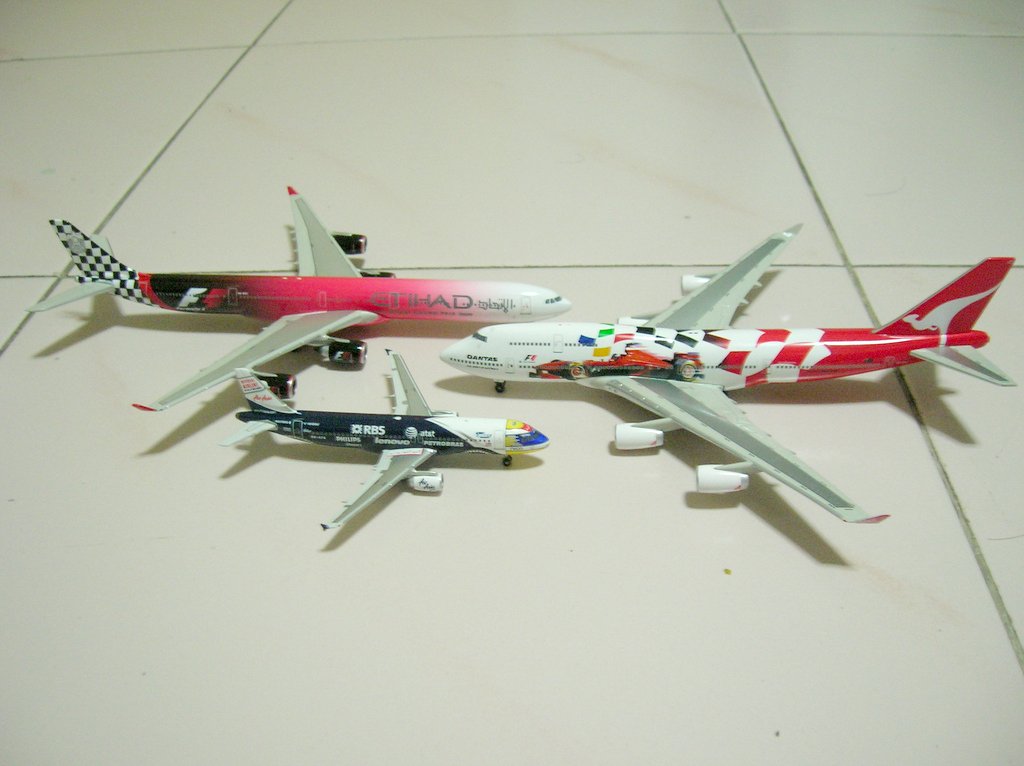A color photograph depicts three model commercial airplanes of varying sizes arranged on a white tile floor with a gray grout grid pattern. Centered in the midline, their tails face outward, and their noses point inward. The planes, reminiscent of metal toys from the '70s or '80s, feature distinctly colorful designs. 

The largest plane, positioned slightly below and facing left, has a white nose transitioning into a body adorned with colorful flag patterns. Its red tail fin prominently features a white kangaroo, indicating it represents Qantas Airlines. 

Above and to the right, the medium-sized plane, facing right, boasts a bright pink fuselage that blends into a black and white checkered tail, with "Etihad" inscribed in gray letters. Its wings are gray with pink tips.

The smallest plane sits below the others, facing inward as well. It has a primarily black body with a yellow nose section highlighted by blue and red details. The lettering "RBS" is visible on its fuselage, along with "Lenovo."

Each plane, detailed and vibrant, rests on an intricately checkered tile floor, making the scene vivid and nostalgic.